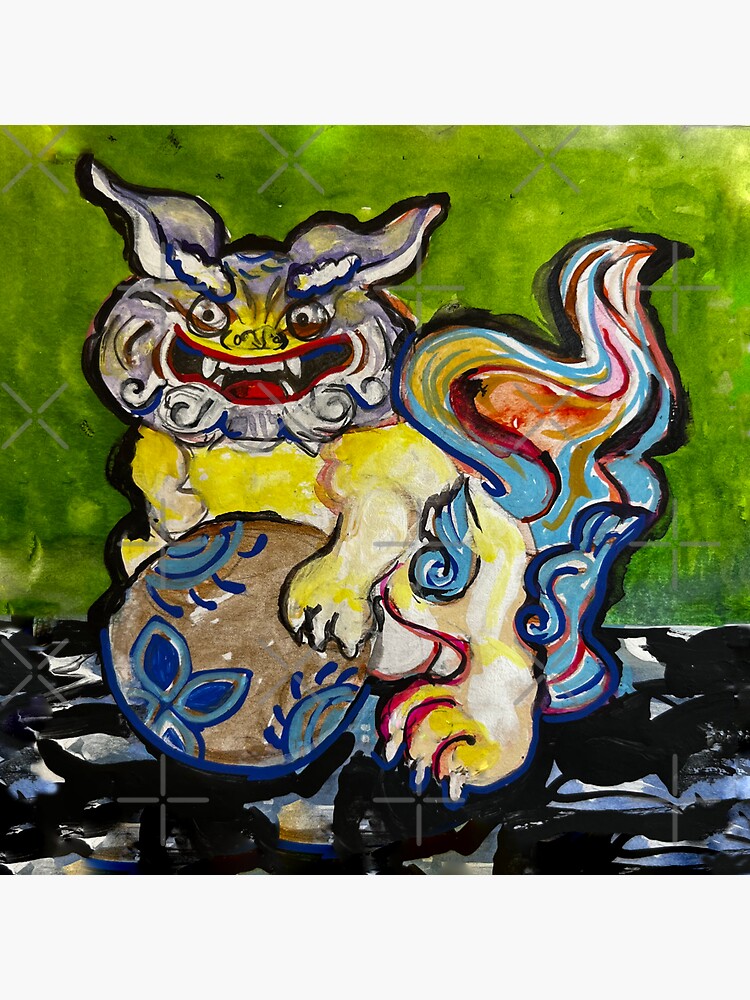The painting vividly portrays a cat-like demon creature centrally positioned against a backdrop of various shades of green. The creature stands on a black surface accentuated with white areas, simulating shiny reflections. The figure itself boasts a striking yellow body and a gray head adorned with curly, beard-like fur around its mouth, adding to its menacing appearance. Its face features an evil grin with sharp white teeth and wide, scary eyes, framed by wavy, upright ears. The creature’s eyes are wide and intense, complemented by pronounced white eyebrows. It clutches a spherical ball in its front paws, which appears tan to grayish and is adorned with various symbols resembling flowers and suns. The demon’s multicolored tail exhibits rich hues and brushstrokes of blue, red, pink, maroon, and orange, potentially giving the tail a striped appearance. The creature's overall demeanor, combined with its vibrant and intense palette, evokes an unsettling yet mesmerizing aura.